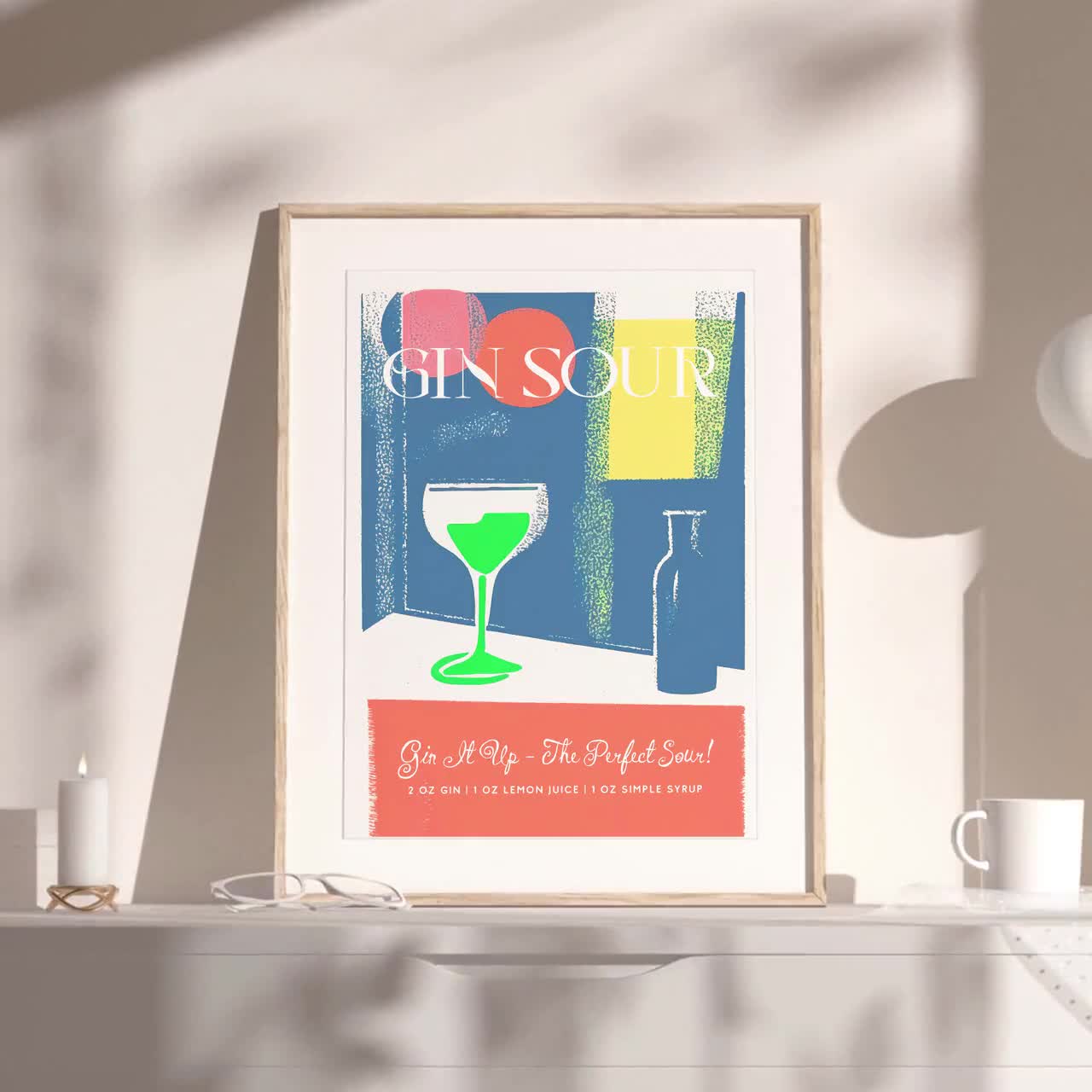In a predominantly white-themed room, a framed print titled "Gin Sour" takes center stage on a white shelf. The print features a martini glass filled with a vibrant lime green liquid, identified as a gin sour cocktail. Beside the glass stands a small bottle of gin. Accents of blue, pink, and red shapes decorate the print, adding a splash of color. The top of the print has "GIN SOUR" written in bold, white, uppercase letters, while below, on a red rectangle, reads "Pin it up the perfect sour" in an elegant script. The recipe is printed beneath: "2 oz gin, 1 oz lemon juice, 1 oz simple syrup" in block letters. The artwork is framed with a natural wood finish and surrounded by a white mat. Surrounding the print on the white shelf are a brass-held white candle on the left, white-rimmed reading glasses in front, and a white mug to the right, blending seamlessly into the minimalist aesthetic of the room.